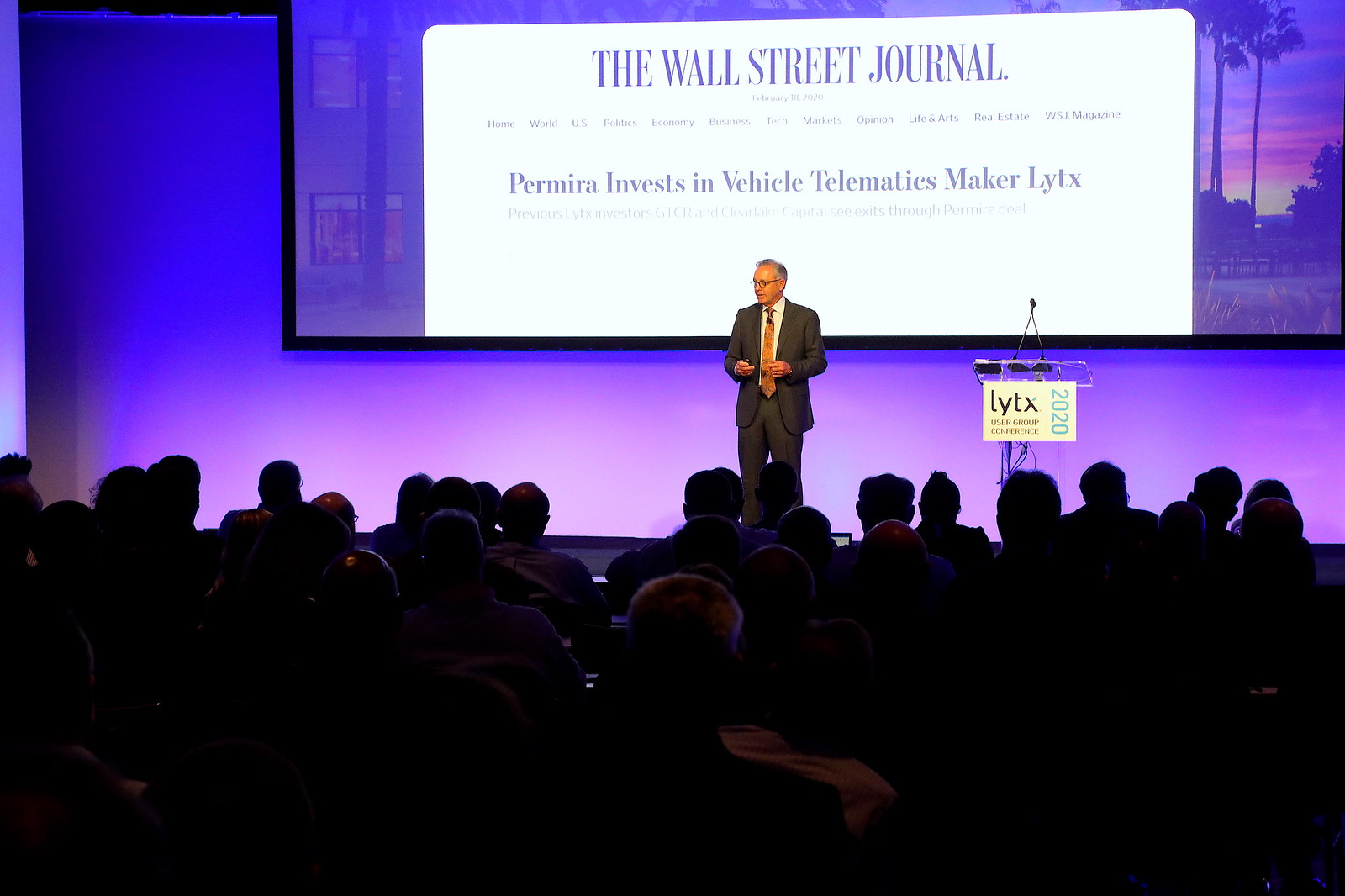The image features a man standing at the center of a stage, addressing a large audience in an auditorium. The man is wearing a gray business suit with a white collared shirt and an orange patterned tie. Silhouettes of the audience and their heads can be seen from the back, with the dimly-lit room suggesting an indoor setting. Behind the speaker, a large screen displays a projection with the words "The Wall Street Journal" in light purple letters on a white background. Below the title, a headline reads, "Permira invests in vehicle telematics maker Lytx." There is a podium to the speaker's right, adorned with a white board that has "LYTX" written in lowercase letters and a light blue "2020" date with smaller text beneath it. The scene is illuminated in shades of black, gray, purple, dark purple, blue, white, and yellow colors, indicating that it is likely during a presentation. To the right of the text on the screen are images that include palm trees and a sunset in hues of yellow and pink.